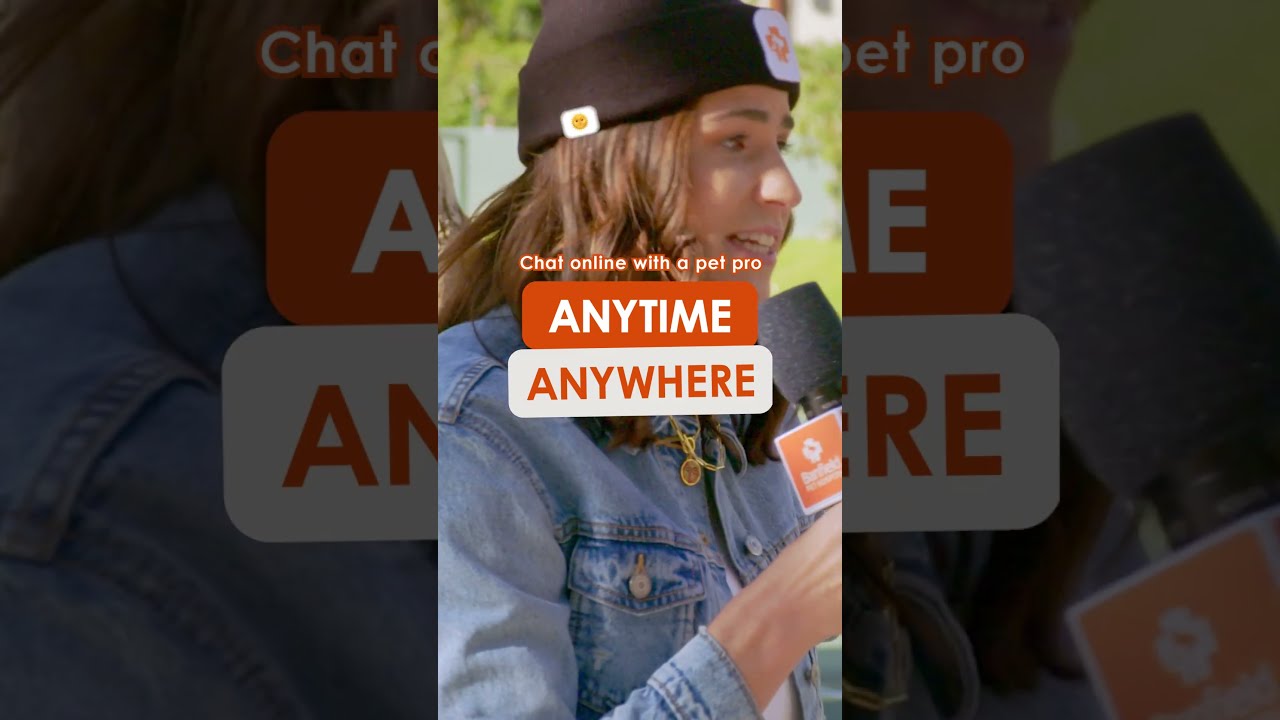The image features a young woman with a lighter skin complexion and long, reddish-brown hair, holding a black microphone adorned with a small orange and white square logo. She is wearing a denim jacket over a white shirt and a black beanie that bears the same orange logo as the microphone. The backdrop of the scene is outdoors, possibly on a street, indicated by the natural daytime light. Centered across the image is the text, "Chat online with a pet pro," displayed in white letters with an orange outline. Beneath this, the phrase "Anytime, anywhere" appears, with the word "anytime" in white letters on an orange background and "anywhere" in orange letters on a white background. This setup suggests she might be part of an interview or video segment discussing pet-related topics.